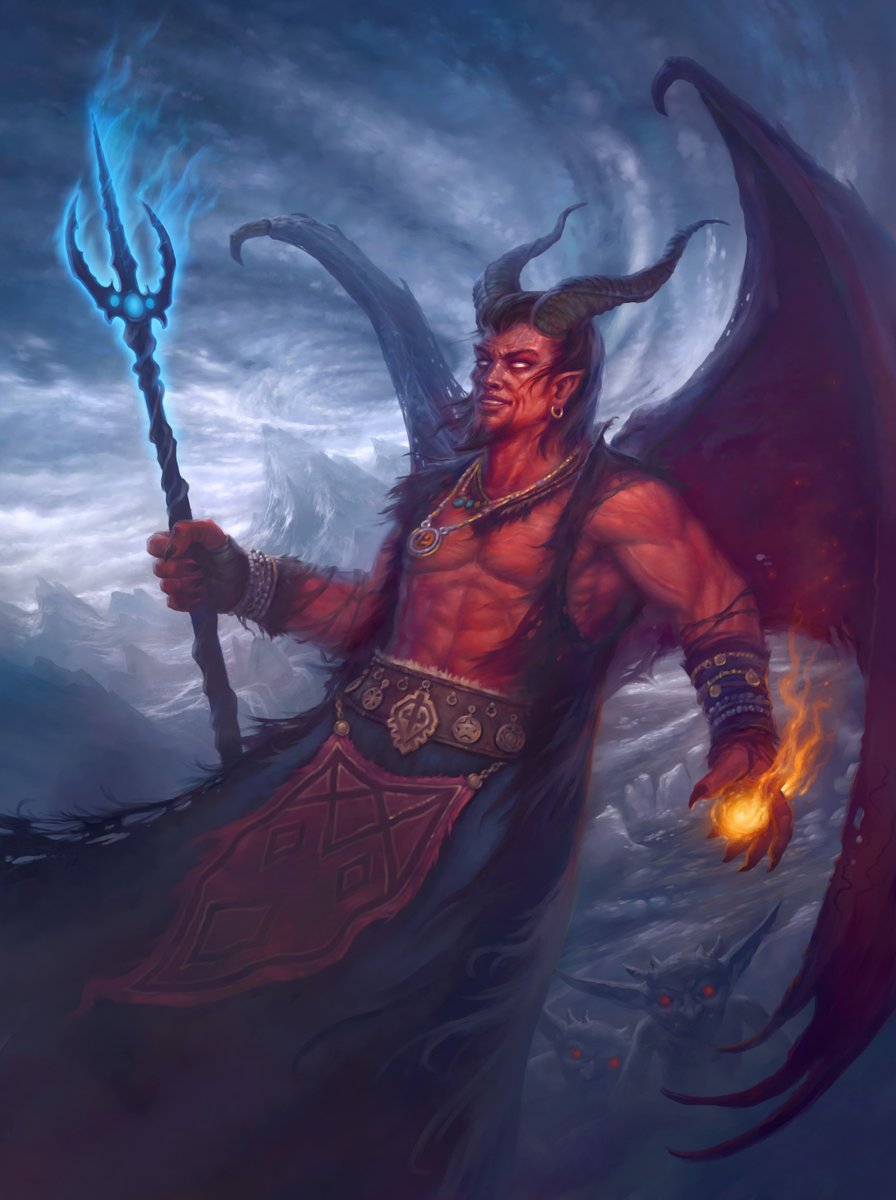This is a fantasy-style digital painting featuring a demon-like figure set against a stormy sky, filled with dark, swirly clouds. The demon has striking red skin, a muscular torso, and wide, black wings with red linings. His imposing presence is accentuated by his large, dark horns, pointy ears, and a goatee on his chin. He sports long brown hair, silver and gold earrings, and a necklace. His piercing white eyes are fixed sternly to the left. In his right hand, he grips a twisted, craggly trident radiating blue energy, while his left hand conjures a fireball. 

The demon is dressed in a distinctive skirt with a blue, triangular banner adorned with gold, and a brown leather belt brimming with jewels and arcane symbols. Two small goblin-like creatures with red eyes lurk in the bottom right corner, adding to the ominous feel. Far in the background, the rugged outline of distant mountains emerges beneath the tempestuous sky, enhancing the otherworldly atmosphere of the scene.